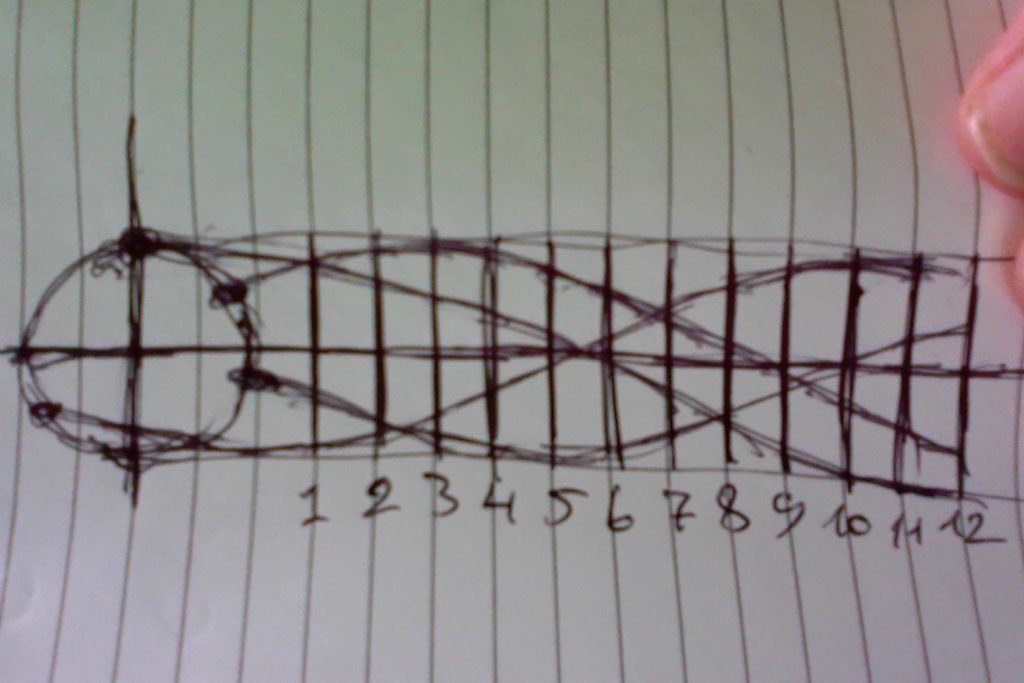The image features a lined piece of paper oriented vertically, with the lines running from the top to the bottom. In the upper right-hand corner, there is a partial view of someone's fingers – one clearly visible and a bit of a second finger. On the left-hand side of the paper, there is a prominent circle intersected by a vertical black line. Another horizontal black line extends from this circle across the entire width of the paper, reaching the right edge. Within this section, several black circles, some oblong in shape, dot the area. Beneath the horizontal line, numbers ranging sequentially from 1 to 12 are printed. Additionally, the paper features thicker black lines accentuating some of the regular lines, complemented by curved black lines that originate from the oblong shapes near the left circle and extend towards the number 12 on the right-hand side.